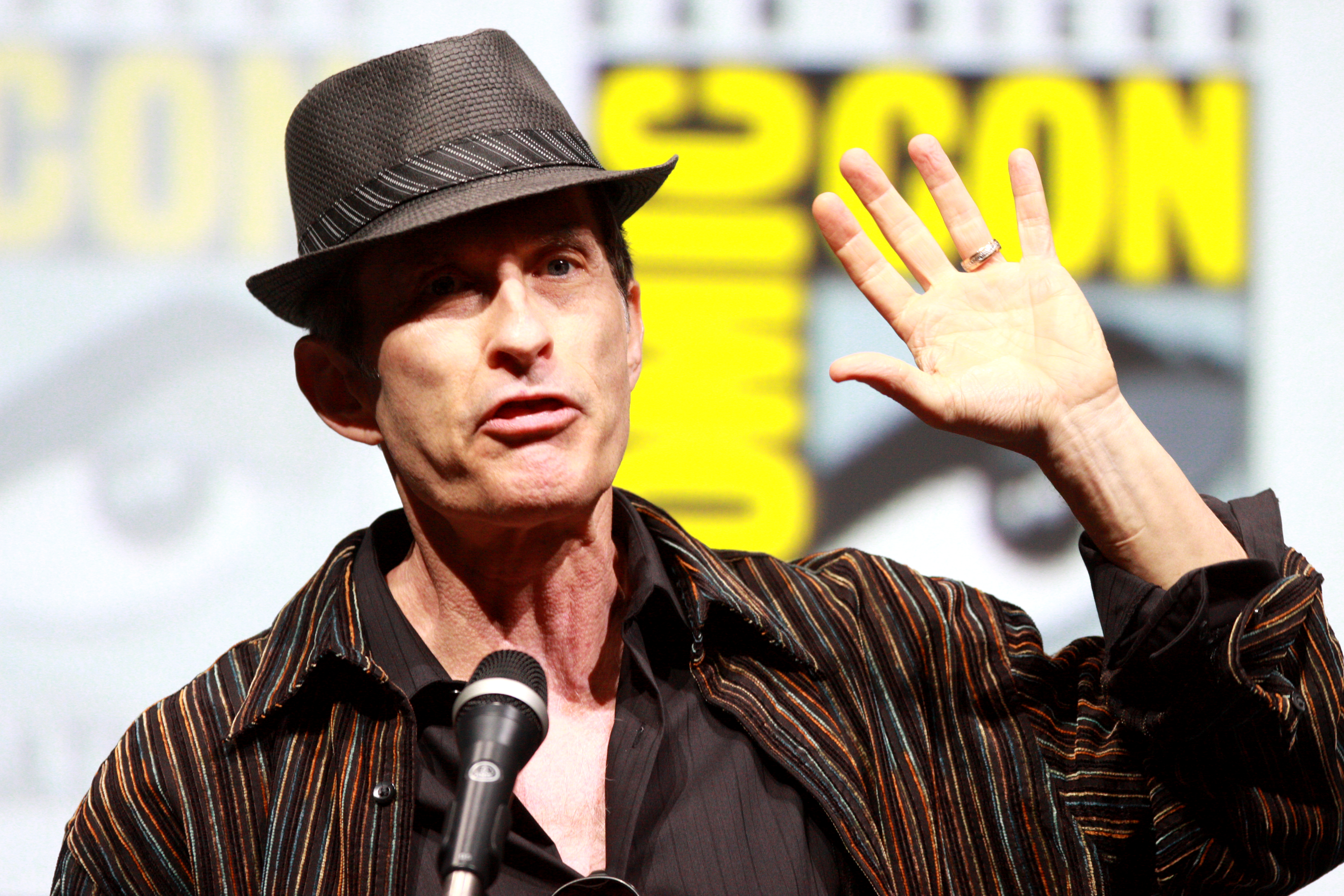The image features a male actor, approximately 50 years old, at Comic-Con, identifiable by the blurry Comic-Con logo with yellow letters visible in the background. He is dressed in a distinctive outfit, including a dark-colored fedora with a striped band around the base, and a layered ensemble consisting of a solid brown undershirt beneath a loosely fitted, dark, striped shirt showcasing blue, red, and black hues. The actor is in mid-speech, holding a microphone in his left hand, and has his right hand raised with an open palm, prominently displaying a ring on his ring finger. His expression appears neutral, neither happy nor sad.